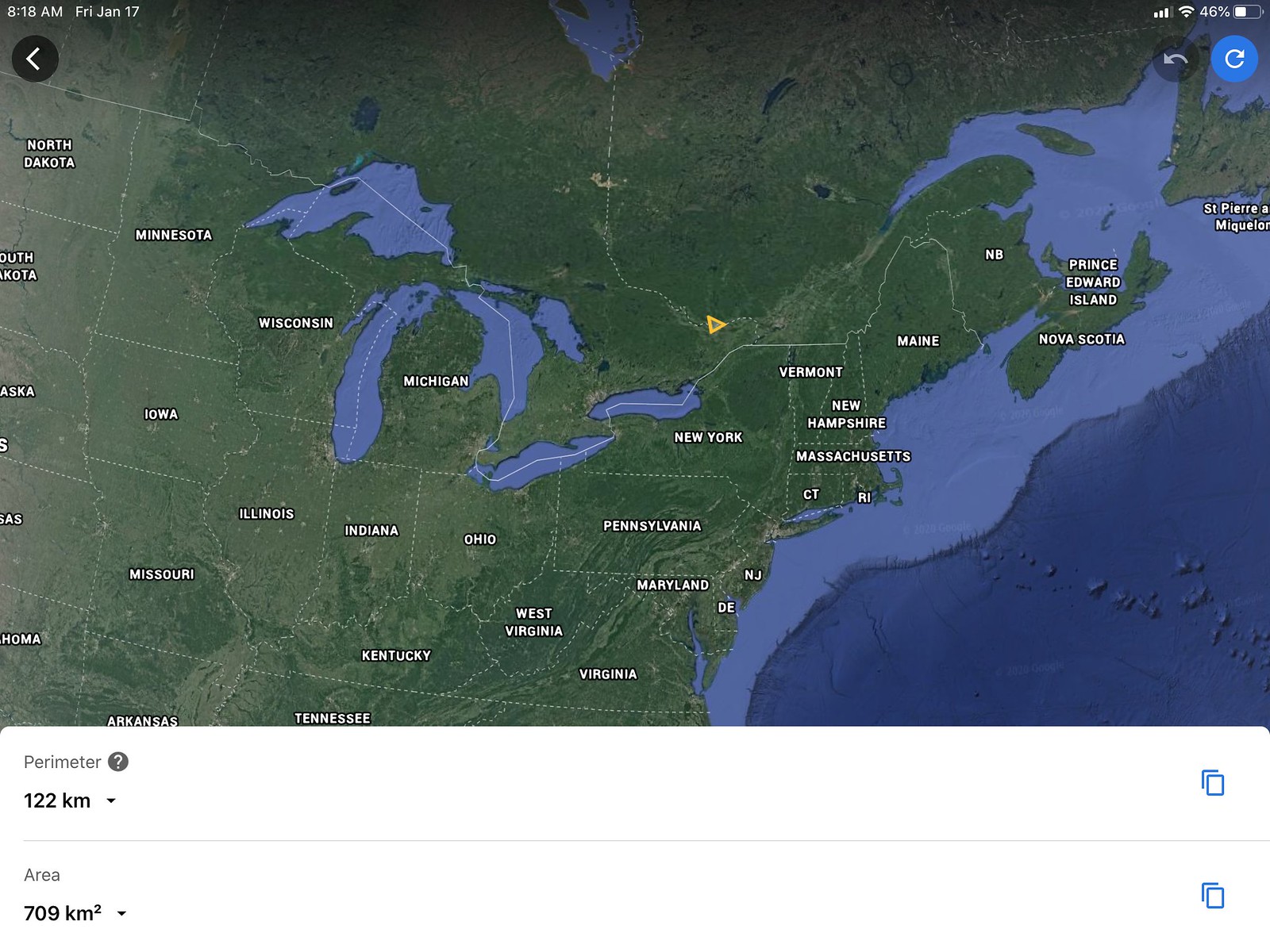This photograph showcases a detailed map highlighting the middle to northeastern regions of the United States, along with portions of Canada towards the top. The land areas on the map are depicted in a vibrant green hue, and the individual states in the United States and provinces in Canada are demarcated with white dotted lines. The international boundary separating the United States and Canada is represented by solid white lines, making it distinctly recognizable.

Several geographic locations are labeled in crisp white text, offering clear identification of key areas. Bodies of water are illustrated with a soothing light blue color, with a deeper shade of blue present in the bottom right corner, possibly indicating a larger water body like an ocean or a significant lake.

Beneath the main mapped area, there is an annotation reading "perimeter 122 kilometers, area 709 kilometers squared," providing specific measurements of the highlighted region's size and boundary length. The meticulous detailing and color usage allow for easy differentiation between various regions and natural features.